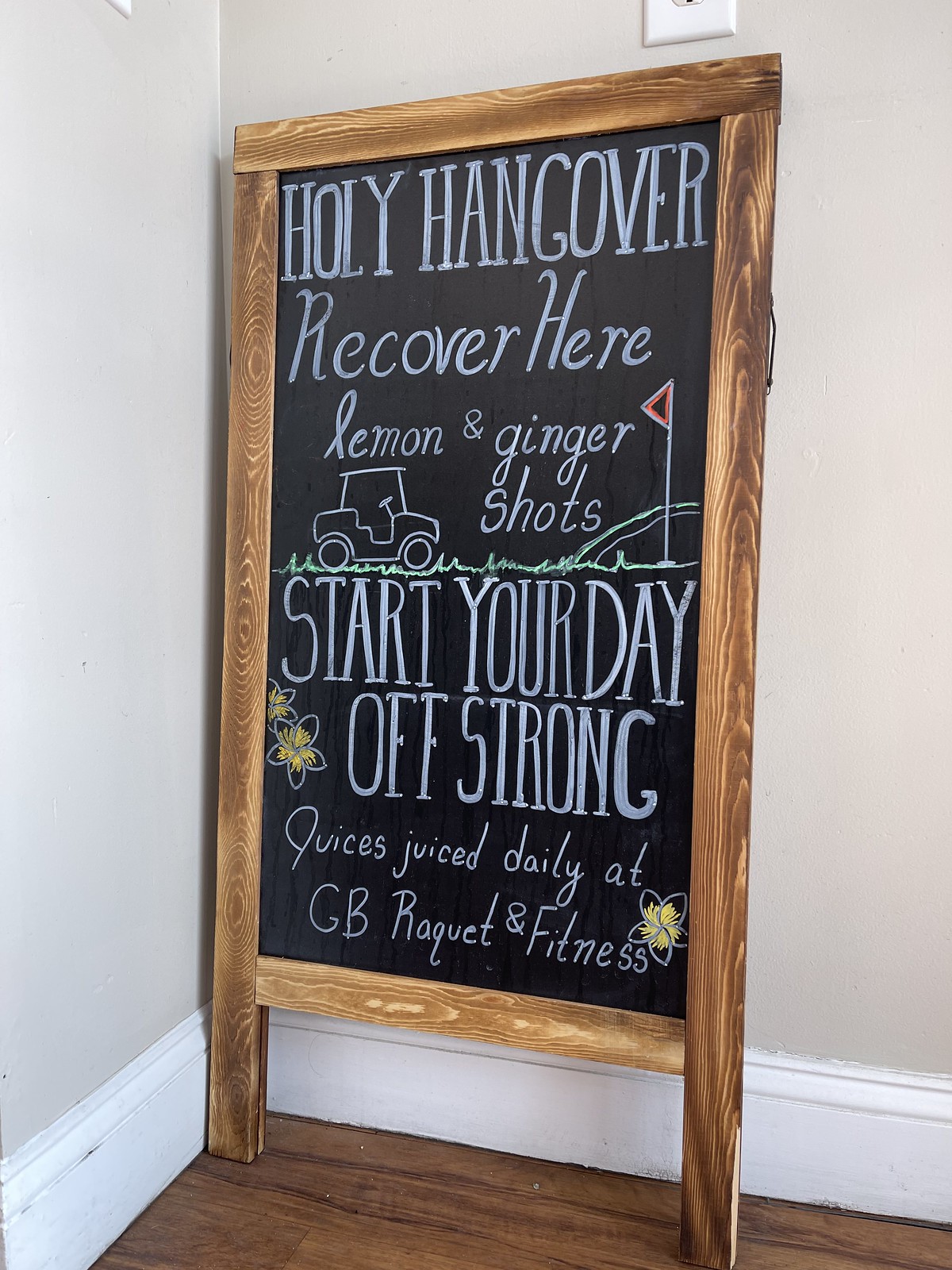The photograph captures a detailed scene of a black chalkboard with a wooden frame, leaning against a light beige wall in the corner of a room with white baseboards and a dark brown wood floor. The chalkboard, rectangular in shape and slightly taller than it is wide, is propped up on the floor with its left and right sides extending beyond the bottom for stability. At the top of the chalkboard in bold white chalk, the text reads "HOLY HANGOVER". Beneath it, also in white chalk, it says "RECOVER HERE". Below this, written in cursive, the message continues with "Lemon and Ginger Shots". Artistically drawn in the middle of the board is a simplistic line drawing of a golf green featuring green grass, a red hole-in-one flag on the right, and a basic golf cart on the left. Underneath the golf imagery, the chalkboard encourages with "Start Your Day Off Strong" in bold white lettering. Further down, it states "Juice this juice daily at GB Racket and Fitness". Near the bottom of the board, three star-shaped flowers in yellowish-orange chalk complete the decorative elements. Additionally, an electrical outlet is visible just above the top of the frame.